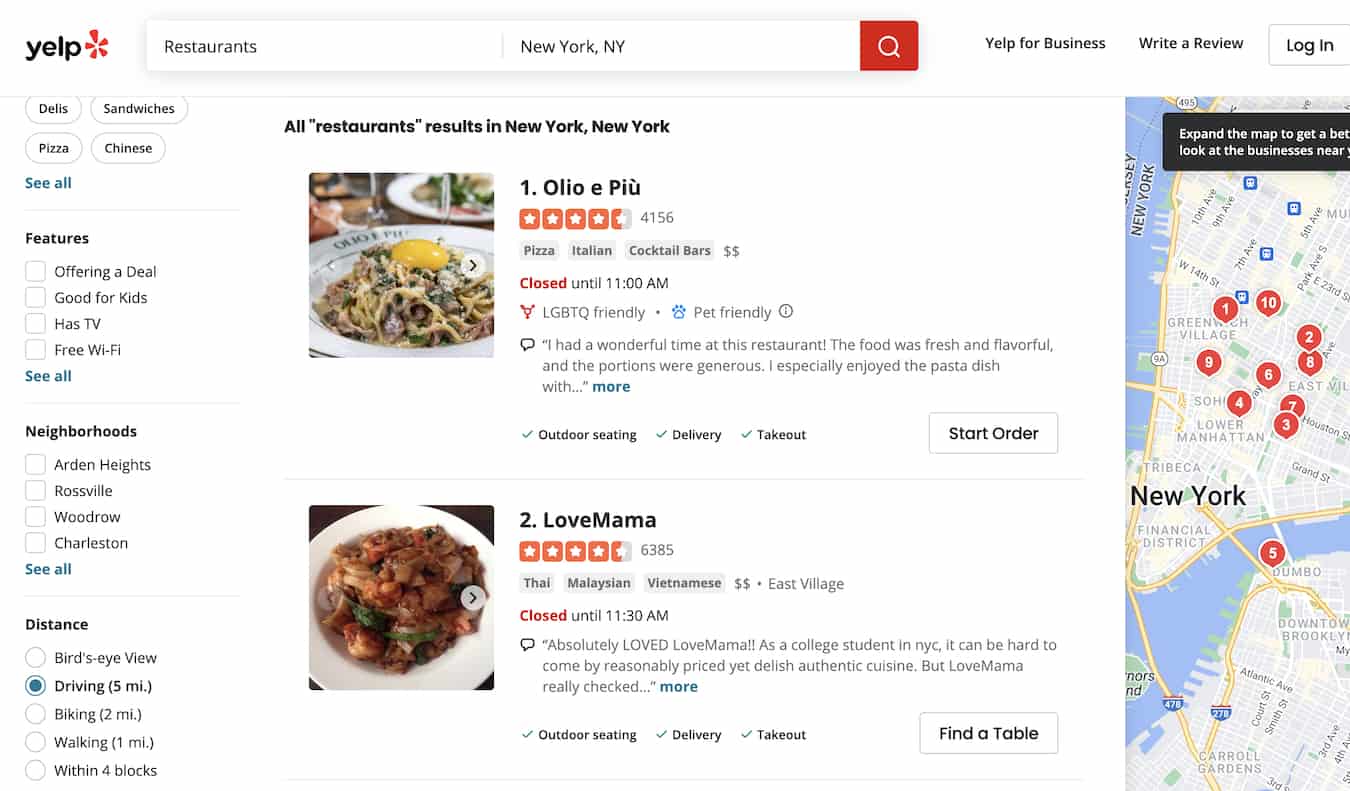This image is a screenshot from the Yelp website. In the top left corner, the familiar Yelp logo is displayed in black lowercase letters next to their iconic red flower emblem. Below the logo, there is a search box with placeholders for "restaurants" and "New York, New York," along with a red search button featuring a magnifying glass icon. Adjacent to the search box, options in black text include "Yelp for Business," "Write a Review," and a login box.

On the left-hand side, there are four clickable bubbles labeled "Delis," "Sandwiches," "Pizza," and "Chinese," with a blue link below that reads "See All." Further down, features are listed with corresponding checkboxes: "Offering a Deal," "Good for Kids," "Has TV," and "Free Wi-Fi." Neighborhood options for browsing include "Arden Heights," "Rossville," "Woodrow," and "Charleston," also selectable via checkboxes. Additionally, a distance filter includes five circles labeled "Bird's Eye View," "Driving (5 miles)," "Biking (2 miles)," "Walking (1 mile)," and "Within 4 Blocks," with "Driving (5 miles)" marked by a blue dot.

In the center of the image, results for "All Restaurants" in New York, New York are displayed. The first featured restaurant is "Olio e Più," which boasts 4.5 stars from 4,156 ratings. This establishment offers Pizza, Italian cuisine, and Cocktail Bars, and is noted as being LGBTQ-friendly and pet-friendly. It is currently closed and will reopen at 11:00 AM. The second establishment, "Love Mama," also has 4.5 stars from 6,385 ratings and serves Thai, Malaysian, and Vietnamese food in the East Village. It is noted for outdoor seating, delivery, and takeout, and is currently closed until 11:30 AM.

On the right-hand side of the image, there is a map of New York City highlighting various locations corresponding to the search results.